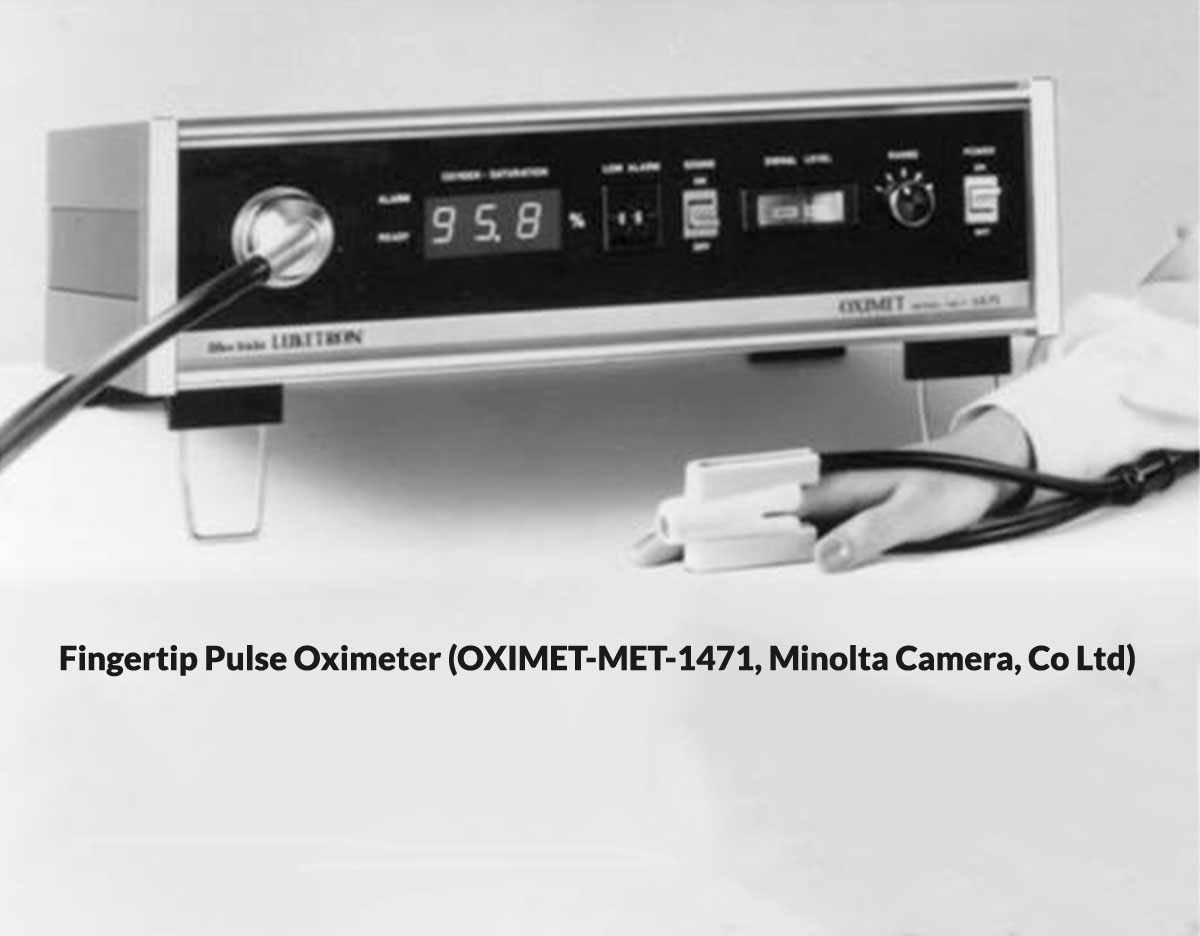This vintage black and white advertisement features a large, oblong, silver-and-black device identified as a "Fingertip Pulse Oximeter Oximet-Met-1471," manufactured by Minolta Camera Co. Ltd. The machine, angled up on wire legs, boasts a display reading "95.8" for oxygen levels and is accompanied by numerous switches, buttons, and a dial with numbers. To the right, a woman in a white shirt rests her hand on a table, with her finger inserted into the plastic oximeter sensor, connected by a black cord. The caption at the bottom of the ad reads: "Finger Pulse Oximeter Oximet-Met-1471 Minolta Camera Co. Ltd.," highlighting the product’s model and manufacturer. The overall appearance and design suggest it's from the early 1960s or 1950s.